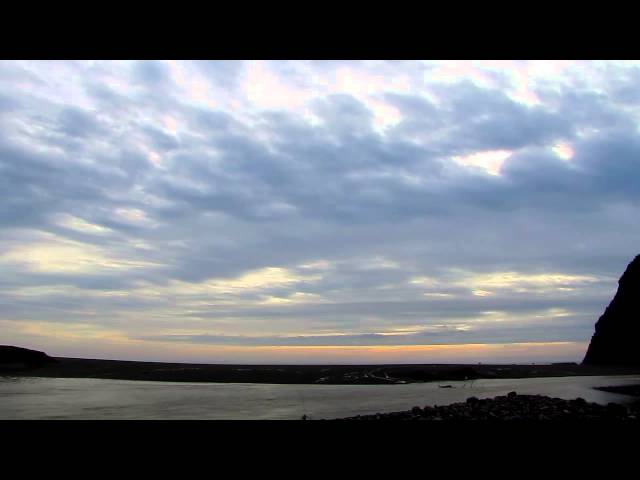This image, captured on an older camera or mobile phone, evokes a sense of nostalgia with its vintage aesthetics. Dominating the scene is a serene view of the sea, framed by two masses of land. The foreground consists of a landmass shrouded in darkness, almost black in color. Flanking the image are two black strips—one at the top and one at the bottom—giving the picture a bordered, almost framed appearance.

The sky captures a stunning transition, with hues blending from deep blues to rich oranges, suggesting the magical moments of either sunrise or sunset. To the right, a shadowy mountain adds to the composition's depth, its details obscured by the dim light. The image has a textured surface, with several parts appearing rough or ruffled, possibly due to the imperfections of the older technology used to take it.

In the far corner, a large beacon makes a faint appearance, challenging the viewer's eyes to distinguish its form amidst the darkened landscape. Overall, the image exudes a moody, enigmatic quality, where the lack of sharp details adds to its charm.